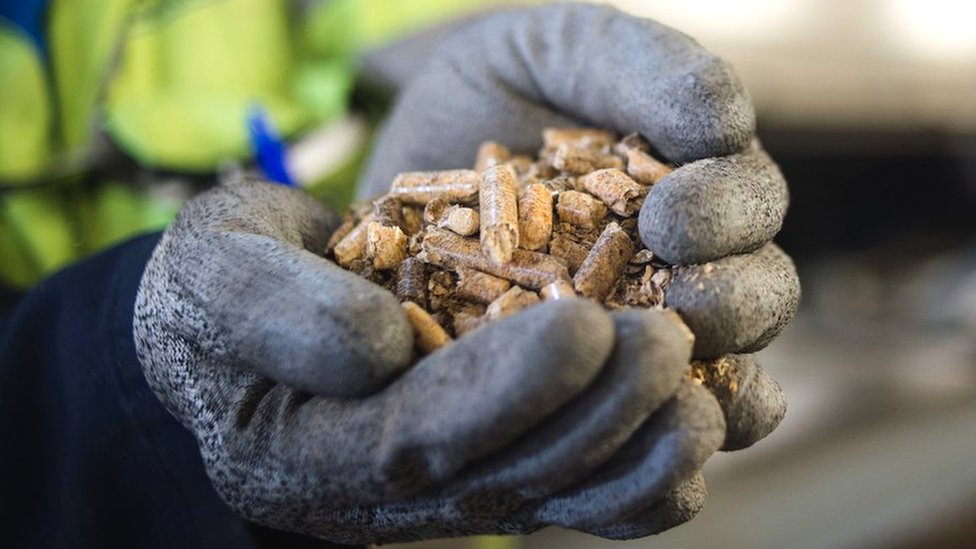The photograph showcases a detailed close-up of gloved hands holding a small pile of light brown, cylindrical wood pellets, some of which are broken into smaller pieces. The gloves appear industrial, dark gray with a special coating on the palms and fingers for added durability. The individual is likely a construction worker, evidenced by the out-of-focus neon yellow-green safety jacket visible in the background. Additional hints of a dark blue long-sleeved shirt are seen beneath the jacket. The background includes blurred white and black shapes, contributing to the industrial setting. The hands are cupped together, cradling the wood pellets, which resemble compressed bits of wood or gravel, adding texture and focus to the image.